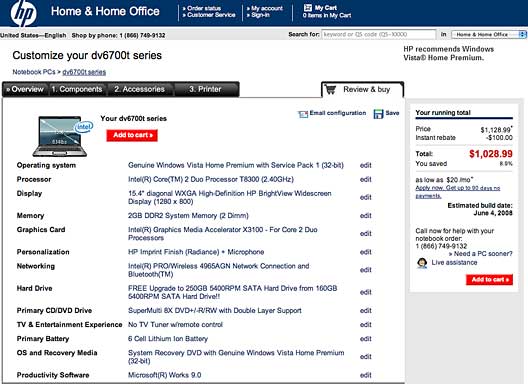The screenshot captured from the HP website features the customization page for the HP DV6700T series notebook. The top part of the page showcases the recognizable HP logo in white and blue, along with navigation options for 'Order', 'Customer Service', 'My Account', 'Sign In', and 'My Cart'.

Under the main section, the customization process for the DV6700T series begins. The notebook category is clearly indicated. Tabs for 'Overview', 'Components', 'Accessories', and 'Printers' are prominently shown in black. An image of a generic-looking laptop is displayed alongside details for configuring the notebook.

The specified configuration includes a genuine Windows Vista Home Premium with Service Pack 1, 32-bit operating system. The chosen processor is an Intel Core 2 Duo. The display size is a 15.4-inch diagonal screen. For memory, the system boasts 2GB DDR2. The graphics are powered by an Intel Graphics Media Accelerator X3100, and the notebook has an HP imprint finish microphone.

The hard drive is a 250GB 5400 RPM SATA, offered as a free upgrade. The primary DVD drive is a SuperMulti 6 DVD. No TV tuner or additional tuner was selected. The battery is a 6-cell lithium-ion. The productivity software included is Microsoft Works 9.0.

The total price for this configuration is listed at $1,028.99. Notably, the build date of this particular configuration would have been June 4th, 2008, indicating that the screenshot is quite dated.